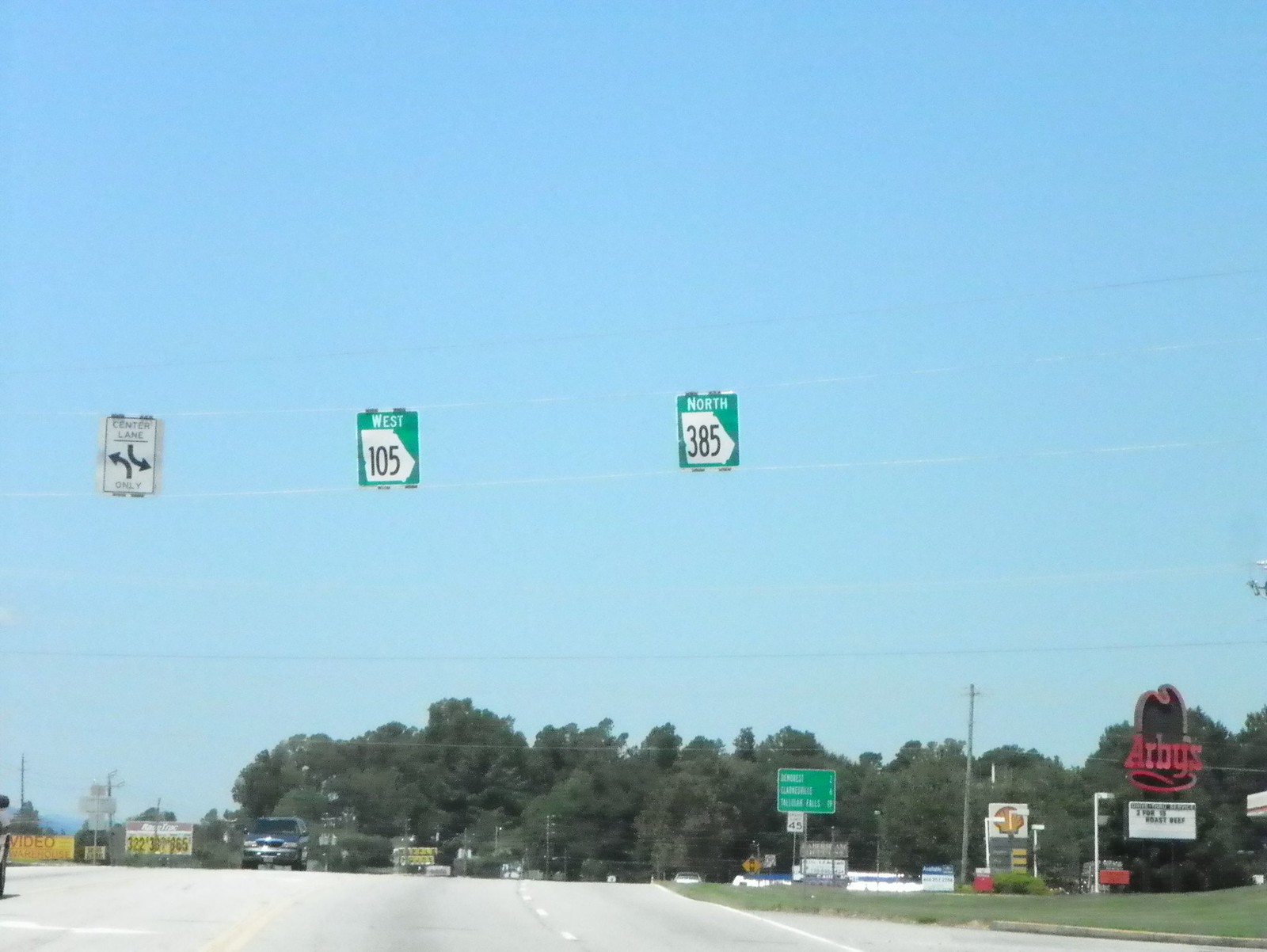The photo captures a wide expanse of blue, cloudless sky above a busy highway scene. Dominating the middle of the frame, hanging on wires, are three signs: a white directional sign with curving arrows indicating a center lane, a green sign featuring "West 105" within an odd, arrow-shaped state outline, and another green sign marked "North 385" similarly outlined. Below these signs, the highway stretches into the distance, bordered by a row of trees along the horizon.

On the lower right, an Arby's sign and a nearby Shell gas station are prominent landmarks. A green highway exit sign, partially obscured, indicates distances to upcoming locations. To the bottom left, a blue car approaches, traveling towards the camera. Nearby, small signs include a yellow "video" sign in red letters and other yellow-background signage. The road itself has a dividing yellow line, separating the two directions of traffic. Additionally, a 45-mile-per-hour speed limit sign is visible on the right side of the road, emphasizing the traffic flow and speed regulations.